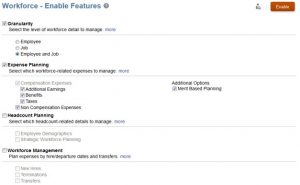A low-resolution screenshot of the "Workforce - Enable Features" page of a software program. The image is blurry with extremely tiny text that makes it difficult to read. At the top, the title "Workforce - Enable Features" is displayed prominently in bold. On the right side of the screen, there is a red rectangular button with text that is illegible due to the poor image quality. Adjacent to the button is a gray icon, which appears to be depicting a person. Beneath this section, there is an outlined list with bullet points and indentations indicating different topics. The main headings in this outline are partially legible, starting with "Granularity," followed by "Expense Planning," "Headcount Planning," and "Workforce Management." Unfortunately, the sub-bullets are too small to read and remain unresolved. Overall, the screenshot provides a general layout of the "Workforce - Enable Features" page but lacks sufficient detail to decipher the full content.